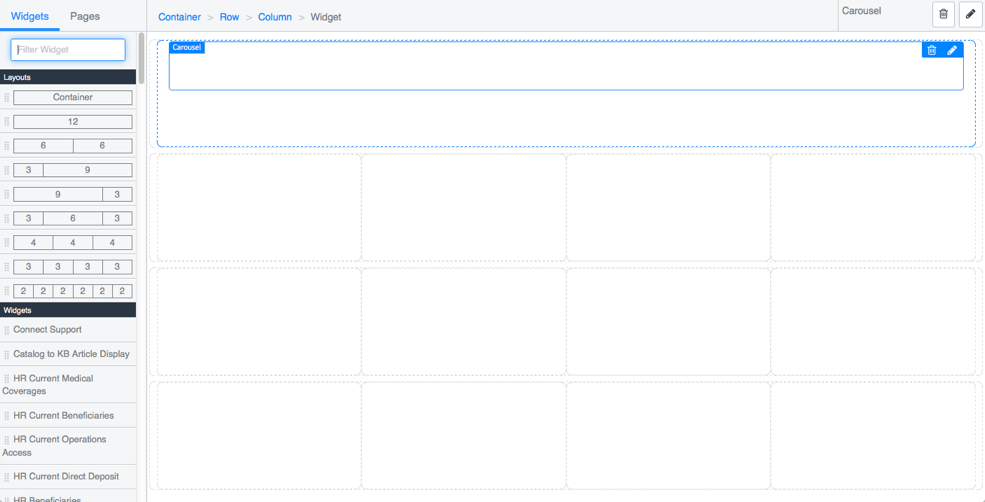The page layout initially appears sparse, dominated by a large white box on the right side, leaving significant empty space. At the top of this box, numerous labels are displayed: "Widgets" (blue and underlined), "Pages" (grey), followed by "Container," "Row," "Column" (all blue), "Widget" (grey), and "Carousel" on the far right, which features an edit pencil and trash can icon. 

On the left side, a dark grey (almost black) vertical strip has the label "Layouts" in white inside a horizontal box. Above this strip, a white box outlined in blue reads "Filter Widget." Below the "Layouts" section are several boxed options: 
1. "Container" 
2. "Twelve" 
3. Two "Six" boxes separated horizontally 
4. A combination of "Three" and "Nine" split horizontally
5. Another similar combination but reversed with "Nine" and "Three"
6. A long rectangle with a line inside 
7. A short square marked "Three"
8. Another rectangle divided into three sections: "Three," "Six," and "Three," separated by vertical lines
9. A rectangular trifecta where each third is marked "Four"
10. A horizontal rectangle split into four parts with "Three" in each section
11. A rectangle with six segments, each labeled "Two"

Beneath the "Layouts" section, there's another dark horizontal box labeled "Widgets" in white. Below that, several operational connections are listed: 
- "Connect Support"
- "Catalog to KB Article Display"
- "HR Current Medical Coverages"
- "HR Current Beneficiaries"
- "HR Current Operations Access"
- "HR Current Direct Deposit"
- "HR Beneficiaries"

The right-hand side also contains a grid comprising 12 small white squares with light grey borders, devoid of any content or text. These elements collectively create a structured yet minimally populated interface.